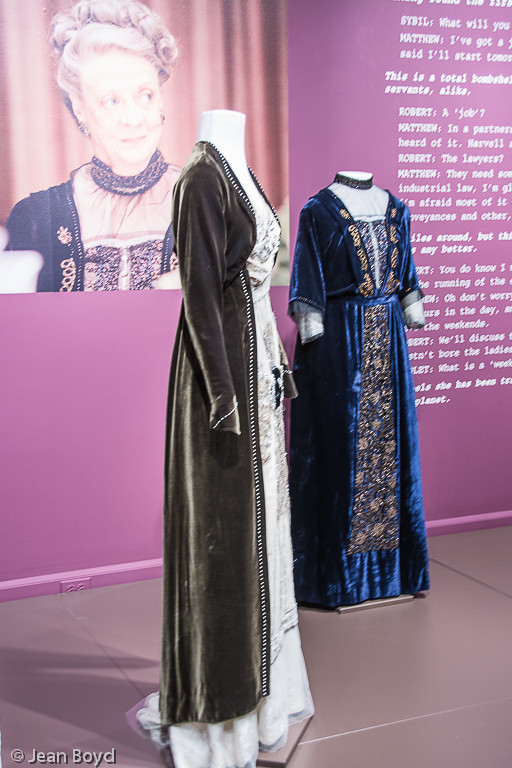The photograph depicts a museum-like display featuring elaborate historical dresses on headless mannequins. In the foreground, the nearest dress is ornately designed in brown and white with intricate patterns, displayed in a side profile. To its right, a blue and gold dress faces forward, showcasing its rich, velvet fabric and detailed embroidery. Both dresses hint at medieval times with their luxurious layers and floral patterns. In the background, a purple wall with partially legible white text frames the scene. The text appears to be a fragmented dialogue reading "Sybil, what will" and "Matthew, I've gotta..." but is largely obscured. Dominating the upper left section of the image is a photograph of an elderly woman, identified as the actress who played Professor McGonagall in Harry Potter. She poses in a black dress with gold accents and a black collar, against a brown backdrop, adding a notable historical and theatrical depth to the display.